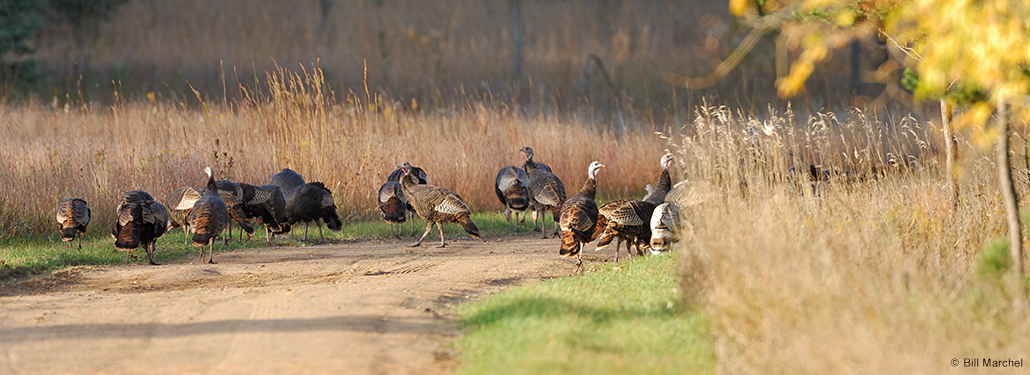This color photograph, taken by Bill Marshall and marked with his copyright in the bottom right corner, captures a daytime scene in a dry, late-season landscape—likely autumn. The horizontal image features a dirt trail cutting across a prairie area, with taller wheat-colored grass and brown weeds growing prominently in the top right corner. In the center of the frame, a flock of approximately 15 wild turkeys, predominantly female, wanders across the path and into the adjacent grassy areas, appearing indifferent to the photographer. The scene is further accentuated by a background that includes yellow-leaved small trees or bushes, blurred towards the top part of the photo, creating a shaded effect against the clearer foreground where the turkeys are foraging and walking in different directions.